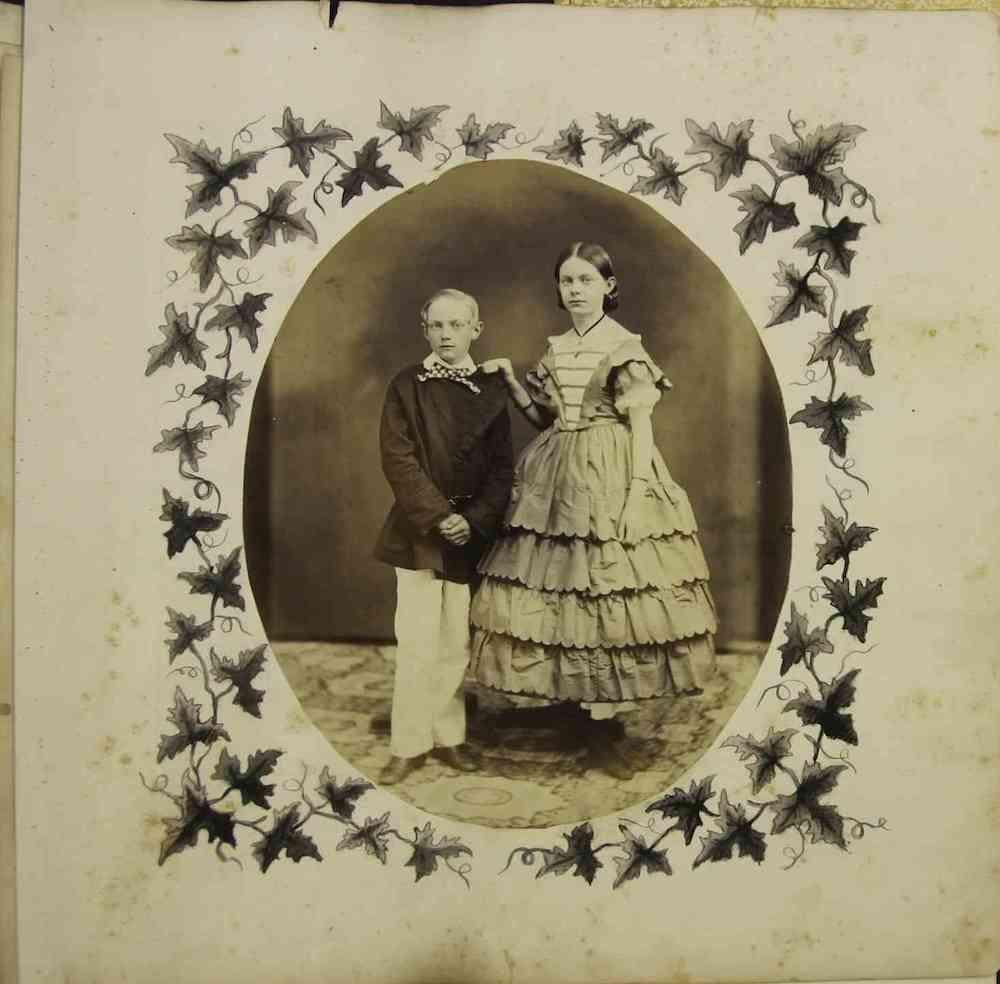This photograph is an antique, likely vintage, image situated within a white square paper mat. The central image is framed by an oval cutout, which is taller than it is wide. This oval is further embellished by a hand-drawn rectangle composed of vine-like ivy, complete with spiraling stems and leaves, adding a touch of organic elegance to the mat's design.

Within the oval, the photograph captures two young individuals, possibly in their pre-teen or early teenage years. The individual on the left is a blonde male, shorter in stature compared to the female on the right. He is dressed in a black jacket paired with white pants, and accessorized with a distinctive bow tie featuring white polka dots.

The female, standing to his side, has short brown hair parted down the middle and tucked neatly behind her ears. She is clothed in a dress characterized by short sleeves and a large, tiered, ruffled skirt, reflecting the fashion sensibilities of the era.

The overall composition of the image, from the delicate ivy border to the detailed attire and expressions of the young subjects, evokes a sense of timeless nostalgia, preserving a moment from the past with intricate beauty.